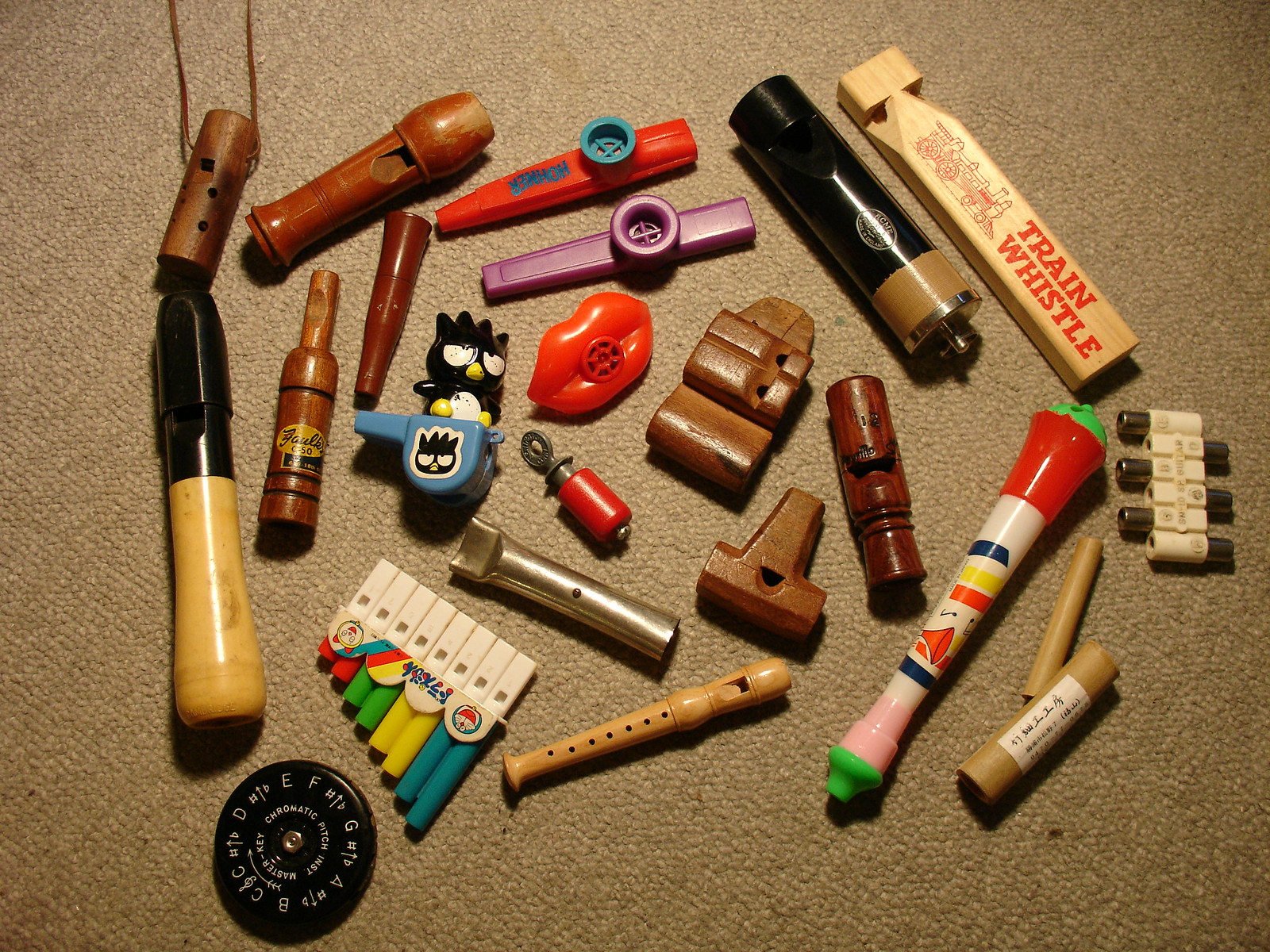The image depicts a collection of various whistles and wind instruments spread out on a light brown, low-fiber carpet, illuminated by light reflecting off their surfaces. Among the assortment are several bright, toy-like kazoos: one with a red body and blue top featuring blue text, and another fully pink. There is a wooden whistle labeled "Train Whistle" in red capital letters with a picture of a train, crafted from smooth, light oak wood. A striking red whistle shaped like a pair of lips and a blue traditional whistle adorned with a sticker of a black bird with spiky hair and a yellow beak stand out as well. 

Additionally, a white multi-whistle features six metal pieces attached to it. A detailed pan flute made of plastic, with each note indicated by a different color (blue, yellow, green, and red), along with a metallic silver tubular whistle, add to the variety. A round black object in the bottom right corner with silver in the center displays the letters A through F in white, resembling a tuning tool. Also present are a brown bottle-like wooden whistle with a yellow logo, a black-and-white tubular object, a T-shaped wooden whistle, and a cylinder-shaped wooden whistle with ridges. An instrument with a green tip transitioning to pink and white, adorned with red, yellow, and blue stripes, and a metal tuning pipe round out the collection. In total, the image captures an intriguing diversity of instruments in different shapes, sizes, and materials, ranging from whimsical toy kazoos to more traditional wood and metal whistles.